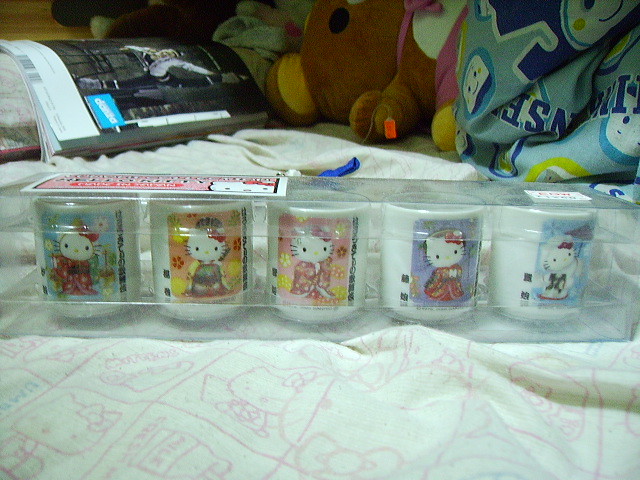The image showcases a display of five Hello Kitty plastic cups, neatly arranged in a clear plastic container. Each cup features a different vertical rectangle design with Hello Kitty depicted in various activities, set against backgrounds in blue, light peach, pink, lavender, and light blue, all adorned with floral elements. The cups are still sealed in their packaging, with Japanese writing visible on the left and right sides of the container. The scene is staged on a bed made with Hello Kitty sheets characterized by a white grid pattern, each box containing different illustrations of Hello Kitty, notably reading a book and holding a milk carton. Additional elements in the background include a blue and white and yellow blanket on the right, an upside-down magazine in the left-hand corner, and the feet of various stuffed animals in the center, with one prominently featuring a red price tag on its paw.